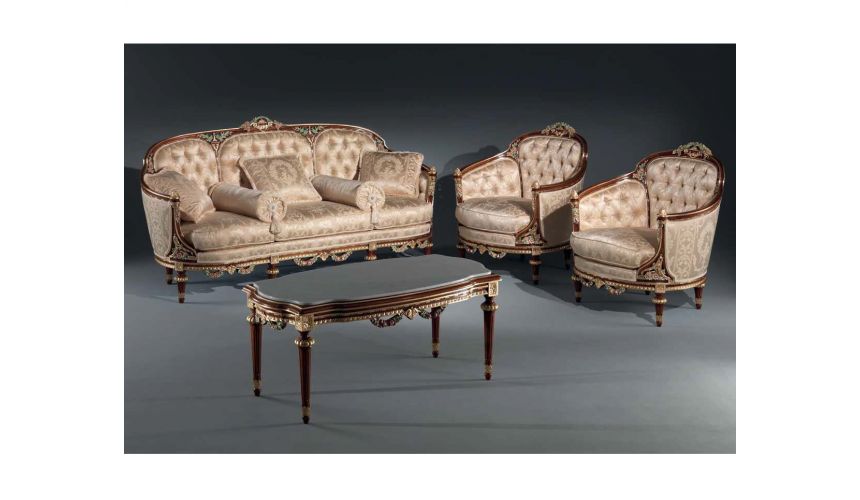The image captures an elegant, 18th-century inspired living room set in a room with a dark grey background and floor, likely designed for a photoshoot or catalogue. The central focus is a regal sofa and two matching easy chairs, all featuring ornate wooden borders with a polished finish, long tapered legs, and luxurious gold-colored upholstery. The sofa, situated in the top left corner of the photo, includes two cylindrical bolsters and three square pillows. To its right, the easy chairs form an L-shape arrangement in the top right corner of the image. Centrally positioned between the seating is a slender, brown wooden coffee table with a grey top and tapered legs. The overall ambiance is one of sophistication and opulence, enhanced by the premium materials and detailed craftsmanship of the furniture set.